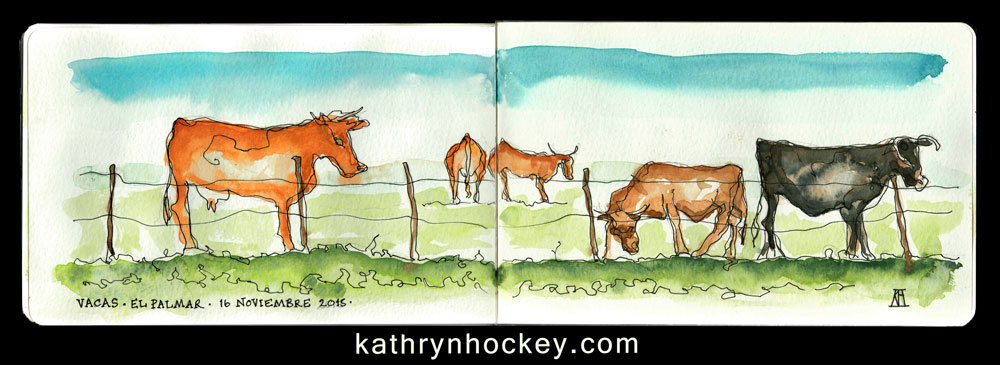This detailed watercolor painting features an idyllic pastoral scene with five cows standing in a green pasture, enclosed by a wire fence supported by brown metal posts. The horizontal artwork is bordered by a black frame that includes the artist's website, katherinehockey.com, at the bottom center. Additionally, the bottom left corner contains the text "Vegas, El Palomar, 16th of November 2015." 

The sky forms a band of turquoise at the top, contrasting with the vibrant greenery of the pasture below. Among the cows, three are positioned in the foreground – two are brown, and one is black with prominent bull horns. Further back, two brown cows appear; one is shown from a rear view while the other is in a side profile. This painting employs a simple line drawing technique that is filled in with watercolor, predominantly using shades of green, brown, black, and blue. A black object is discernible in the bottom right corner, adding to the composition's detail and quality.